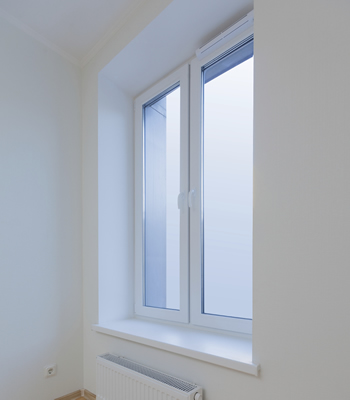This photograph captures the interior of a home, showcasing a predominantly white room with minimal furnishings. The main focus is a large, rectangular window, divided vertically into two panes with handles on each side, allowing for individual or combined opening. The window frame and surrounding walls are painted white, creating a clean, monochromatic aesthetic. Below the window is a small, white gas radiator attached to the wall.

On the left side of the image, there's a wall with white paint and an outlet near the floor, indicative of European design. The floor itself, visible in a small portion of the image, appears to be a tan brown color, possibly with brown baseboards. The surrounding area is devoid of curtains or blinds, adding to the minimalistic feel.

Outside the window, the scene appears overcast, with a white sky suggesting a cloudy day. There is a faint outline of a grey wall or structure to the left, but beyond that, visibility is limited, revealing mostly a bright, cloudy expanse. The ceiling inside the room continues the white theme, contributing to the airy and spacious atmosphere of the photograph.